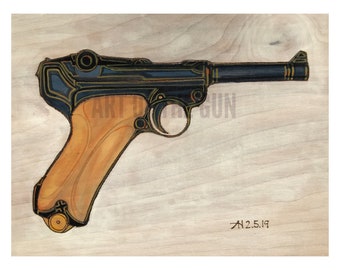This image showcases a detailed piece of artwork featuring an artist's rendering of a gun. The gun, pointing towards the right side, has a brown wooden handle and a black stock, barrel, and trigger adorned with copper or gold trimmings. It is set against a light brown background with a wooden texture, complete with areas resembling wood knots. Overlaying the image is a light gray, bold text that reads "Art of the Gun," partially obscured by the gun itself. In the bottom right corner, the marking "AH2.5.19," likely the artist's initials and the date February 5th, 2019, is inscribed in black. There are no people or additional objects in the image, emphasizing the gun as the central subject of this artistic composition.